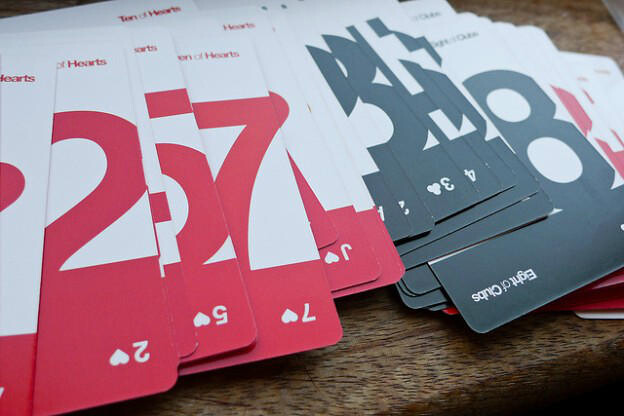A detailed photograph displays a table scattered with several stacks of playing cards, organized by color and suit. These unique cards deviate from traditional playing cards, featuring a minimalist design with a prominent white background and a thick colored banner across the middle. Each card prominently displays its number, which appears to melt into the banner's vibrant hue. The black cards are characterized by a black banner, such as the "8 of Clubs," with the complete card name written out. Similarly, the red cards are adorned with banners in shades of red, such as the "7 of Hearts" and "5 of Hearts." The cards are meticulously grouped by suits — hearts, clubs, diamonds, and spades — forming tall, distinct piles that create a visually striking and organized arrangement on the tabletop.